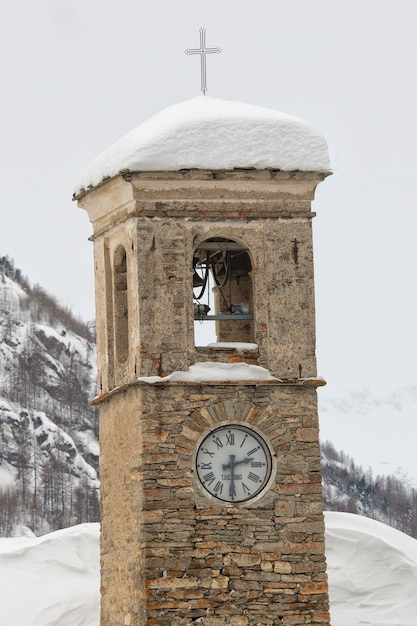The image features a clock tower made of irregularly shaped, stacked stone bricks, prominently displaying a clock with Roman numerals that reads 2:30. The tower, blanketed by approximately 12 inches of snow, has a cross atop the pillar. Midway up the tower, a bell can be seen, hinting at the chime mechanism. The surrounding scenery is a winter wonderland with piles of snow both on top of the tower and all around its base, obscuring any additional structures. In the backdrop, a snow-covered hill or mountain rises, dotted with bare, leafless trees and some dead vegetation poking through the snow. The predominant colors in the image are white, silver, black, gray, and brown, emphasizing the stark winter landscape.